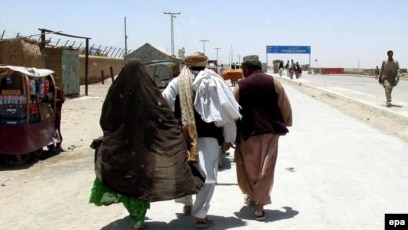In this detailed outdoor photograph, three individuals, possibly refugees or immigrants, are seen walking away from the camera in what appears to be a Middle Eastern setting. The trio, consisting of two men and a woman, are dressed in traditional attire, with the woman adorned in a long black shawl that reaches her ankles, partially obscuring her figure. One of the men wears white pants, a matching white robe, and a tannish brown headscarf, while the other sports loose-fitting light brown pants paired with a dark burgundy vest and a short cap. The group walks along the side of a dirt road littered with junk machinery and wires. To the left, there is a cart or small vehicle, which appears stationary. In the background, a banner marking a border crossing can be seen, flanked by what seem to be soldiers, indicating a checkpoint. Towards the distant right, a blurry figure approaches the camera. Scattered around the border crossing are additional people, evidencing movement and the bleak reality faced by those in the image. The text 'EPA' is also present, adding a possibly political or environmental context to the scene.